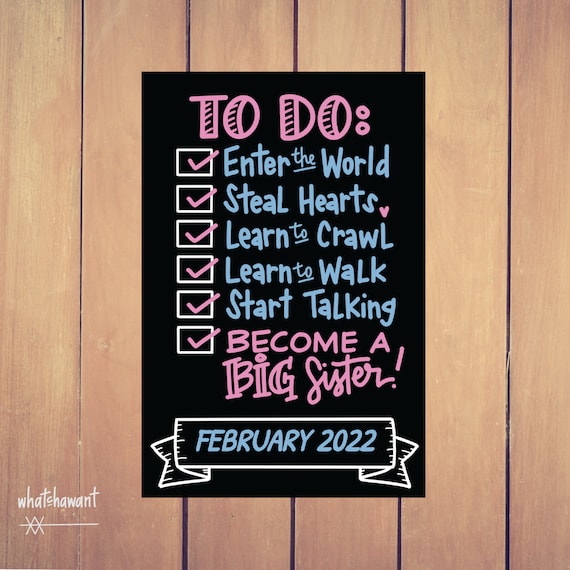A square image showcases a faux wooden panel wall, composed of six vertical slats separated by thin black lines. Centrally mounted on this backdrop is a black poster. At the top of the poster, "TO DO" is prominently displayed in large pink letters. Below this heading is a checklist with blue text and accompanying white boxes checked in pink. The items on the list read: "ENTER THE WORLD," "STEAL HEARTS," "LEARN TO CRAWL," "LEARN TO WALK," "START TALKING," and "BECOME A BIG SISTER." Towards the bottom, a white-bordered banner with black center and blue lettering proclaims "FEBRUARY 2022." In the bottom left corner of the poster, "What's Hawant?" is written in white text, alongside a decoration of two X's crossed by a horizontal line. The pastel hues of purple and blue writing, along with some white drawings, contribute to the poster's visually appealing design.